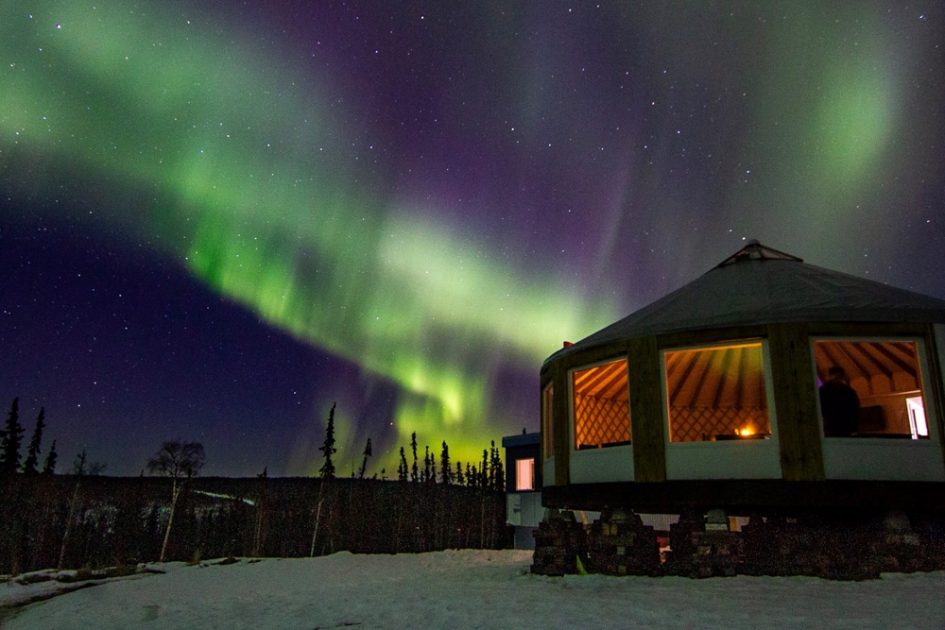This nighttime photo beautifully captures the Northern Lights, or Aurora Borealis, cascading from the sky over a serene campground. The dark sky is vividly illuminated by yellow and green streaks of light descending from the upper right corner, tapering off into a blue expanse with twinkling stars. In the foreground, there's a modern-day yurt with large glass windows, allowing a glimpse into the cozy, well-lit interior. The yurt is either hexagonal or octagonal, supported by sturdy wooden legs. Its ceiling features brown and white stripes, adding a rustic charm. Below, the ground is sandy, with a wooden fence running from the left to the middle of the image, and trees standing tall behind it. The overall scene is a harmonious blend of natural wonder and human comfort.